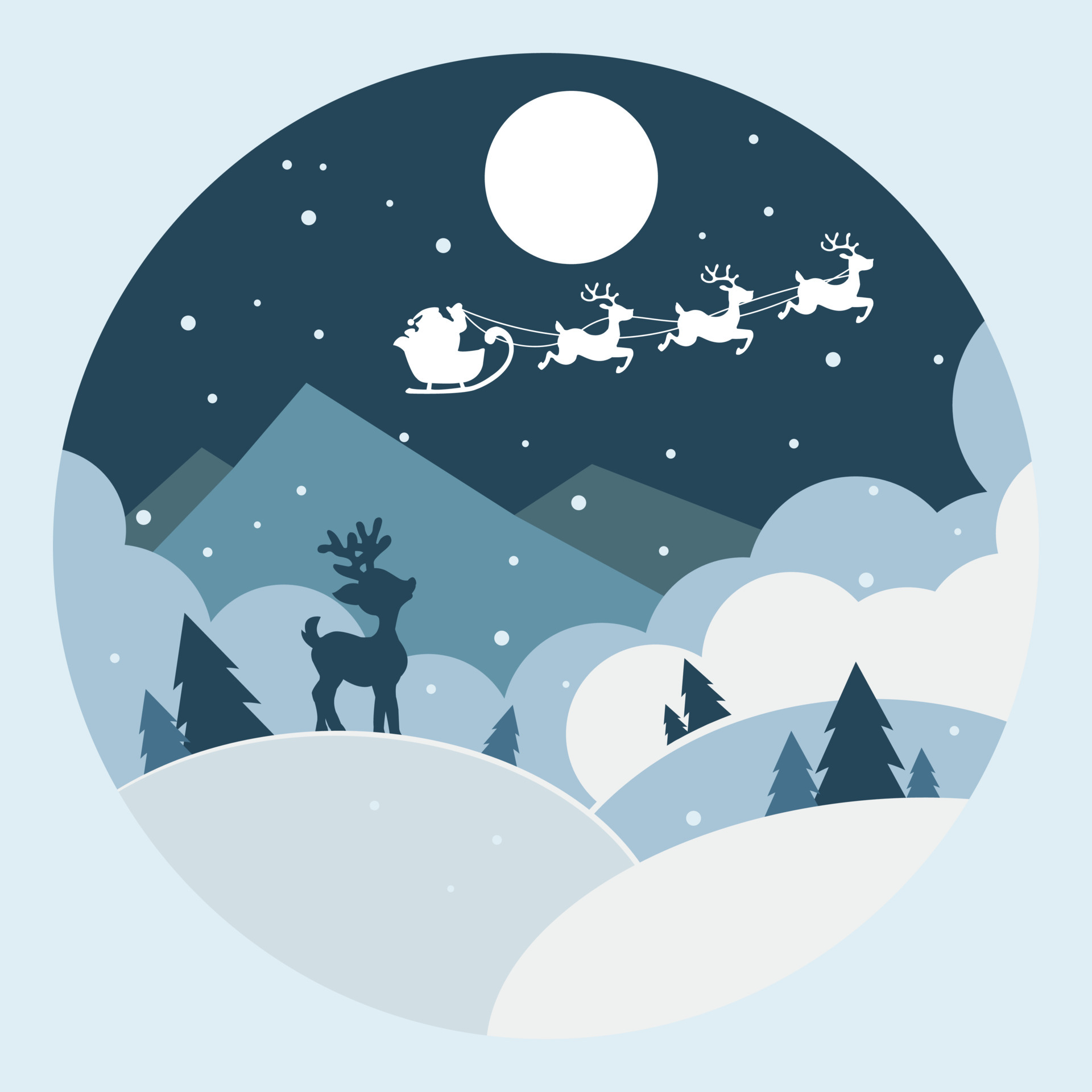This digital illustration depicts a serene winter scene during Christmastime, encased within a circular frame set against a light blue background. Within the circle, a minimalist style is employed using simple shapes and a limited color palette of blues, grays, and whites. The landscape features gently rolling mounds in light blue, gray, and white, evoking snowy hills. Dark blue and blue-gray silhouettes of evergreen trees and a solitary dark navy or teal reindeer, gazing upwards, add depth to the foreground. Three towering mountain peaks, in dark blue and dark gray, rise majestically in the background. The night sky is adorned with a white, circular moon and speckled with white dots resembling falling snow. Hovering above the scene, the white silhouettes of Santa Claus and his sleigh, drawn by three reindeer, soar gracefully. Overall, the illustration conveys a whimsical and tranquil holiday ambiance.